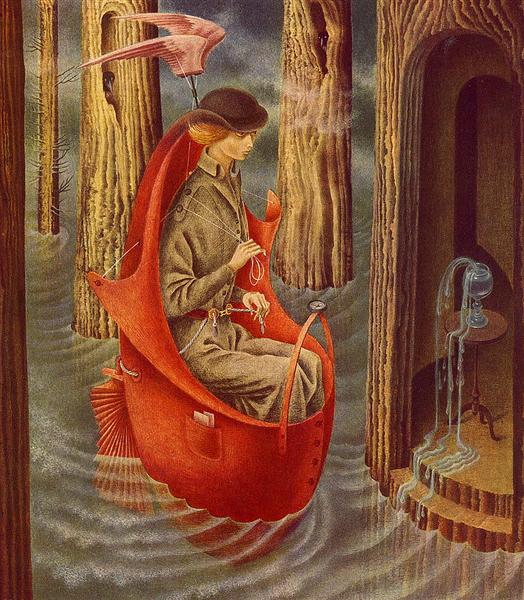In this detailed fantasy illustration, the central figure is seated on a mystical, floating fish-like chair with fin-like gills underneath. The chair, an orangey-red contraption adorned with pockets, buttons, and a compass, appears to be navigated by strings held by the figure. This figure, of indeterminate sex, has an elongated body, exceptionally skeletal hands, a fair complexion, a pointy nose, and tufts of red hair jutting out from under a black hat. Above the chair, pink wing-like appendages, reminiscent of flamingo wings, are also suspended by strings held by the figure.

The scene is set on a body of still water, punctuated by ripples, with eerie, dead trees emerging from it. Three of these trees contain various items within their hollowed trunks: one holds a leaking cup, and two others cradling birds. The water is shrouded in a mist, adding to the haunting atmosphere, and the trees are notably close together. The overall style resembles old artistic coloration with blotchy effects, enhancing the painting's surreal and mystical feel.